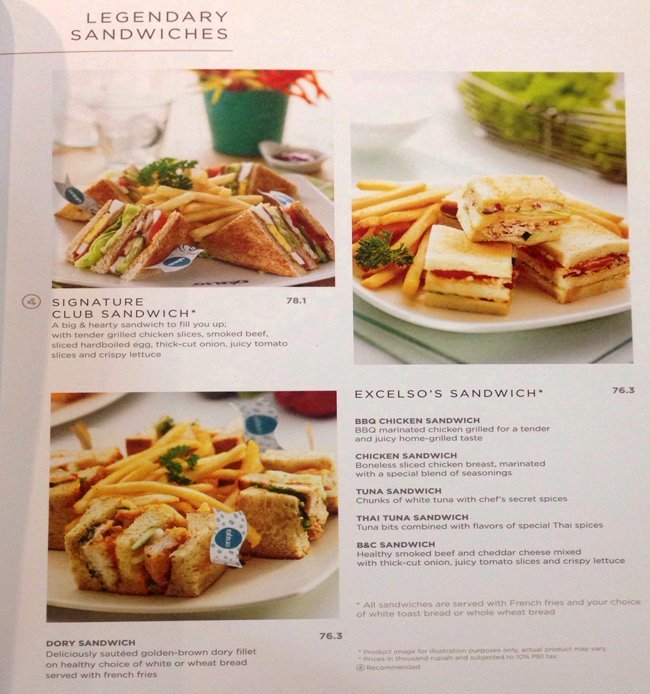The image depicts a detailed menu from an establishment called "Legendary Sandwiches," set against a clean white background. At the top left, it features a large, visually appealing photograph labeled "Signature Club Sandwich" priced at $78.1. This picture shows a plate of several triangular sandwiches brimming with various meats and veggies, arranged around a generous portion of French fries in the center. A dipping sauce is also included, and in the background, a flower pot and see-through drinking cups add a touch of elegance.

Directly below, the "Dory Sandwich" is similarly presented, but the sandwiches here are cut into square shapes, also accompanied by fries. To the right of the top image, a slightly larger photograph displays the "Excelsa Sandwich," priced at $76.3, similar to the Dory Sandwich. This section signifies a variety of sandwich options under the Excelsa category, including Barbecue Chicken Sandwich, Chicken Sandwich, Tuna Sandwich, Thai Tuna Sandwich, and B&C Sandwich. Each sandwich picture emphasizes the freshness and vibrant colors of the ingredients, with toasted bread and an assortment of vegetables contributing to an appetizing and colorful visual.